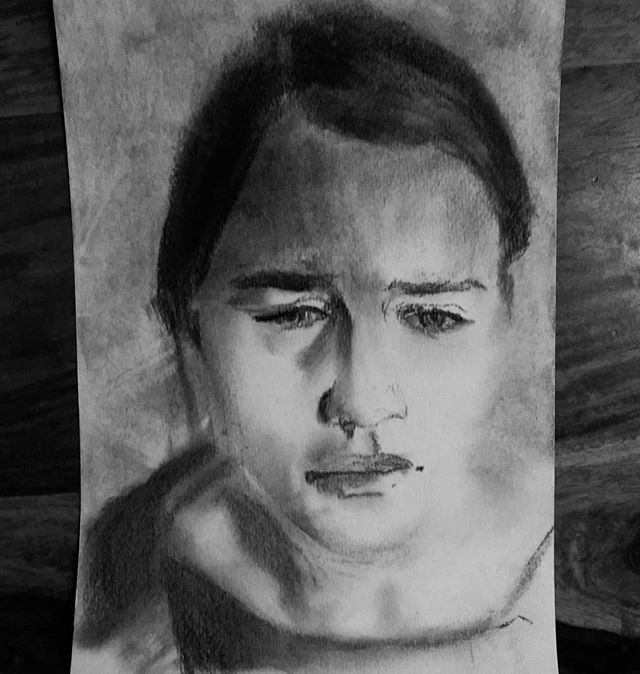This image depicts a meticulously detailed black and white sketch of a person, rendered in a classic style with no color. The sketch reveals the upper torso and face of the subject from a frontal perspective. At the bottom of the sketch, there is a shaded line that transitions into a thicker, darker shaded area on the left side, indicating part of the clothing or body. There is additional shading above this region, while lighter shading appears on the right-hand side, adding depth and dimension to the upper torso.

The face of the subject is intricately detailed, with the lower part remaining predominantly white, while the forehead is extensively shaded in gray. The facial features, including the lips, nose, eyes, and eyebrows, are clearly defined, showcasing the artist's attention to detail. The hair, shaded in black, frames the top of the head, contributing to the overall contrast and structure of the portrait.

The drawing is done on a piece of gray, older-style paper, giving it a vintage feel. The background, visible on both the right and left sides of the paper, features what appears to be a gray wooden table, adding a subtle but complementary element to the composition.